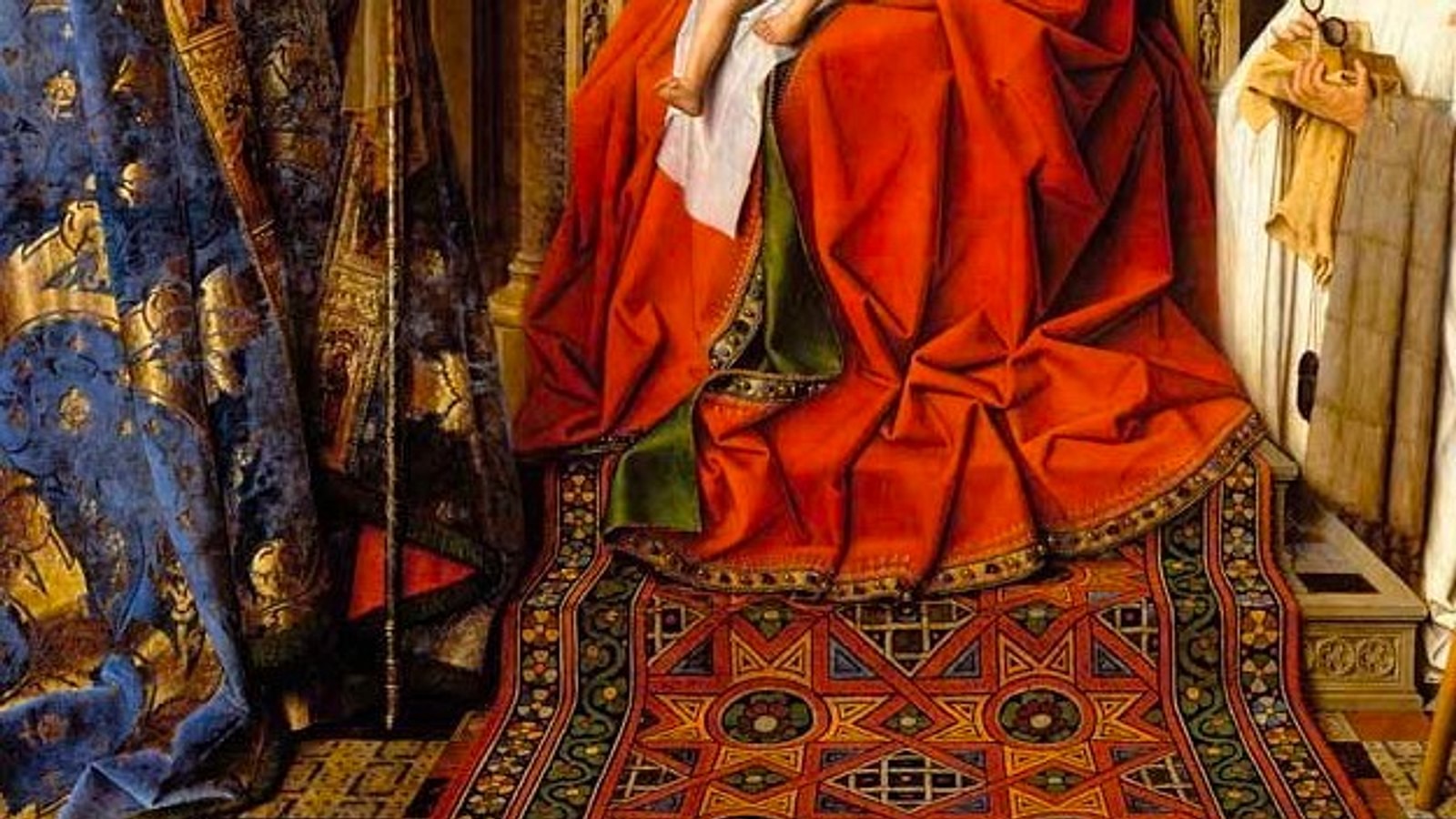The image appears to be a cropped segment of an elaborate artwork, horizontally aligned and rich in detail. On the left side, there are long, ornate drapes or gowns. One is blue with a gold pattern, while another is gold with a dark brown or black pattern. Near these, there is a suggestion of a long metal cane or stick.

In the center of the image, we see the bottom half of a person's gown, orange with brown and gold trim, draping down and touching a red carpet. This carpet features circles, geometric shapes, and by one account, crosses and lines. The person is seated on an elevated platform, likely a throne, with stone stairs partially covered by the aforementioned rug. The throne is described as brown-gold wood with intricate designs.

Additionally, two small baby-like legs are visible at the top middle of the image, creating a focal point along with a small white cloth beneath them. 

On closer examination, just to the right, another set of hands appears to be offering something to the person on the throne, adding to the regal and ceremonial atmosphere of the scene.